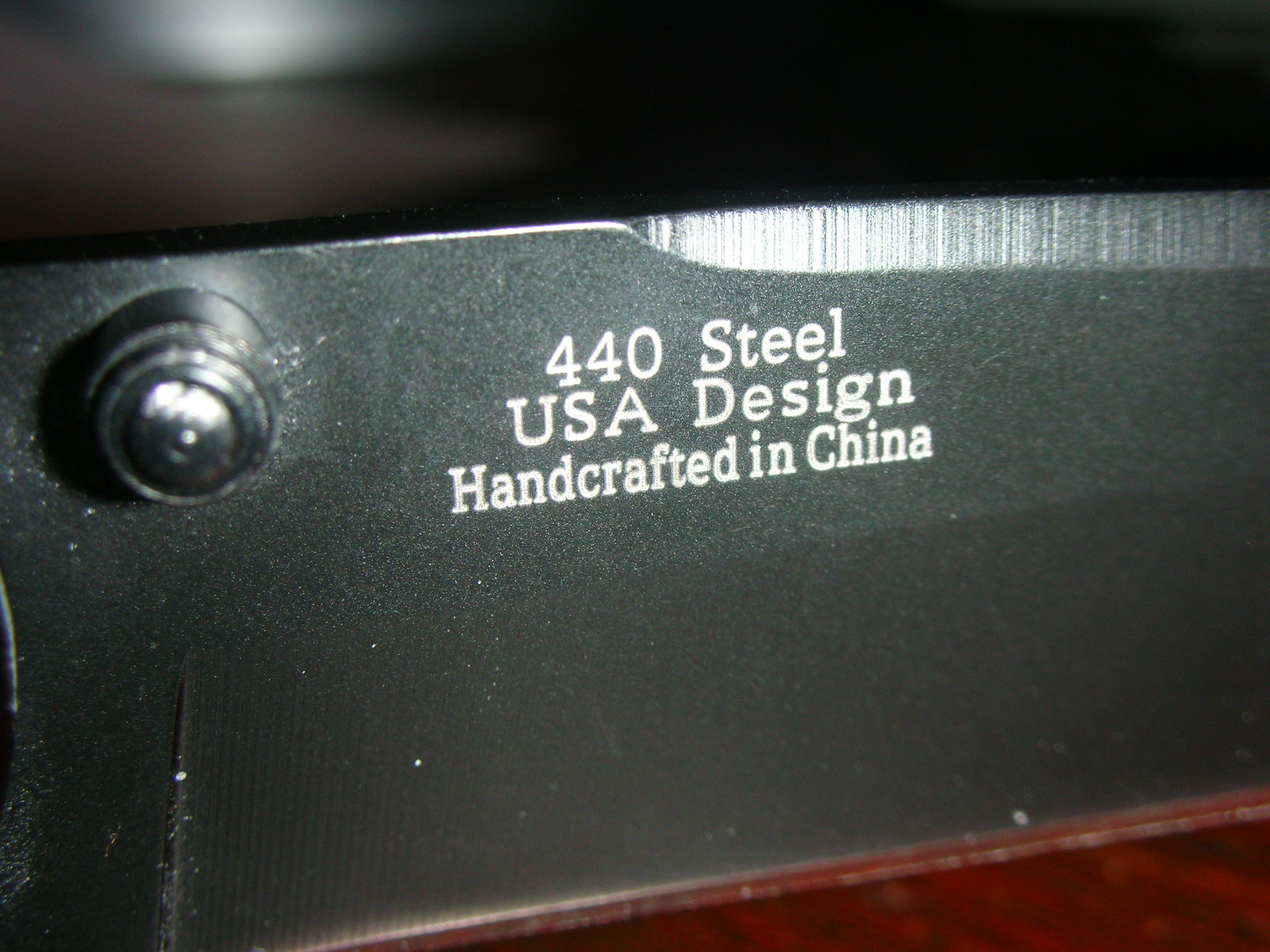The image features a slender, upright metallic object that appears to be a knife. The knife is a thin, gray heather color with a black bolt located near the upper left section. The upper half of the knife is adorned with white lettering that states, "440 steel, USA design, handcrafted in China." The design itself transitions from a uniform gray heather color to increasingly silver tones, accentuated by granular lines that run horizontally. Near the lower left corner, there is a noticeable straight bulge, adding to the intricate detailing of the knife's surface.